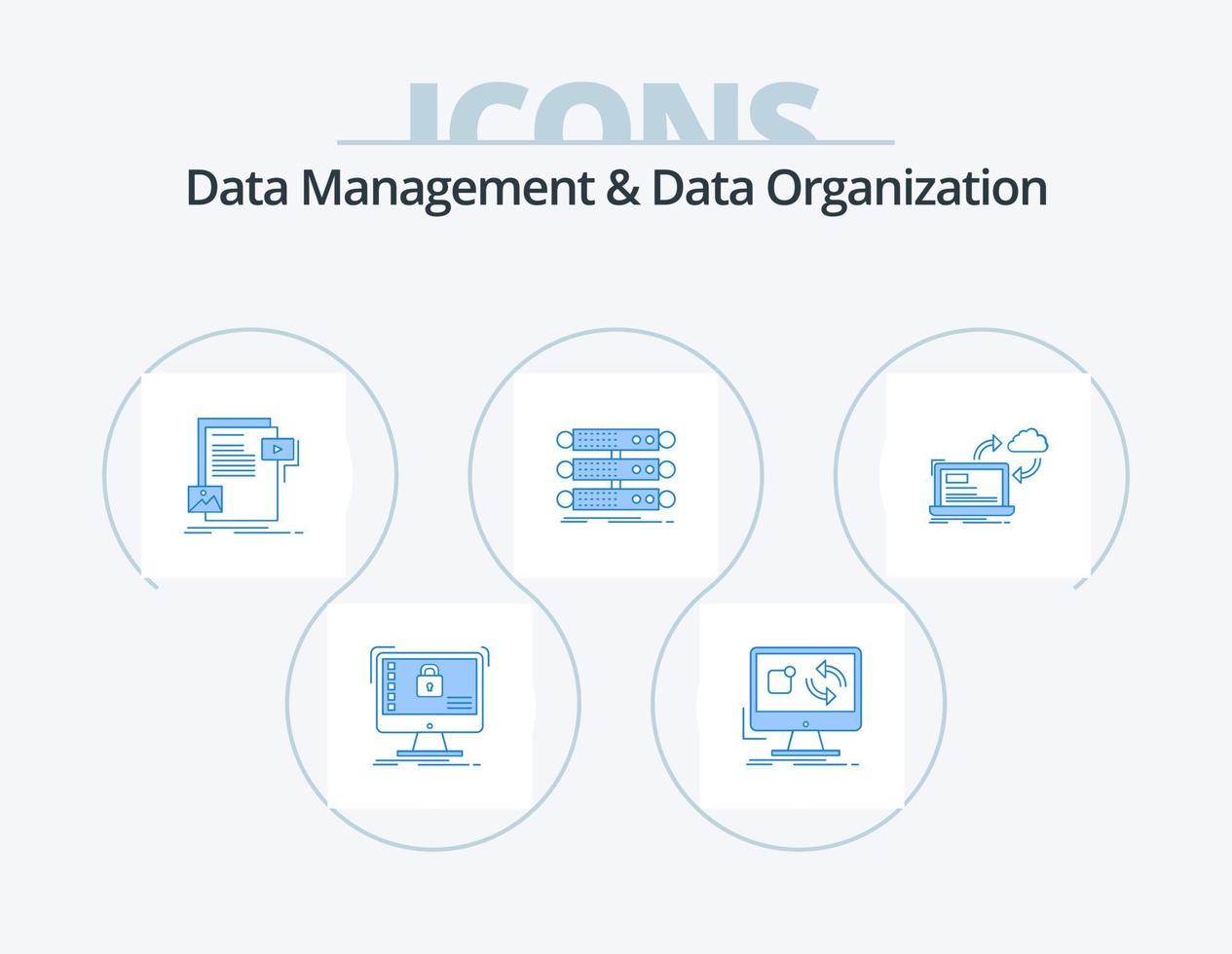The image features an off-white background with a central, square layout. At the top, in a stylized grayish-blue font, the word "ICONS" is displayed in capital letters and centered, but only the top half of the letters are visible due to an underline that bisects them horizontally. Below this, in smaller black font, are the words "Data Management" and "Data Organization." 

The lower section contains five white-bordered squares arranged in a staggered, zigzag pattern. Each square contains an icon illustrating different aspects of data management and organization. The icons include:
- A web page
- A computer with a lock symbol indicating security
- Data servers representing data storage
- A computer with a transfer icon symbolizing data transfer
- A laptop linked to a cloud, denoting cloud storage.

These squares are interconnected by a curved, circular arrow that flows from left to right, visually linking the concepts together.